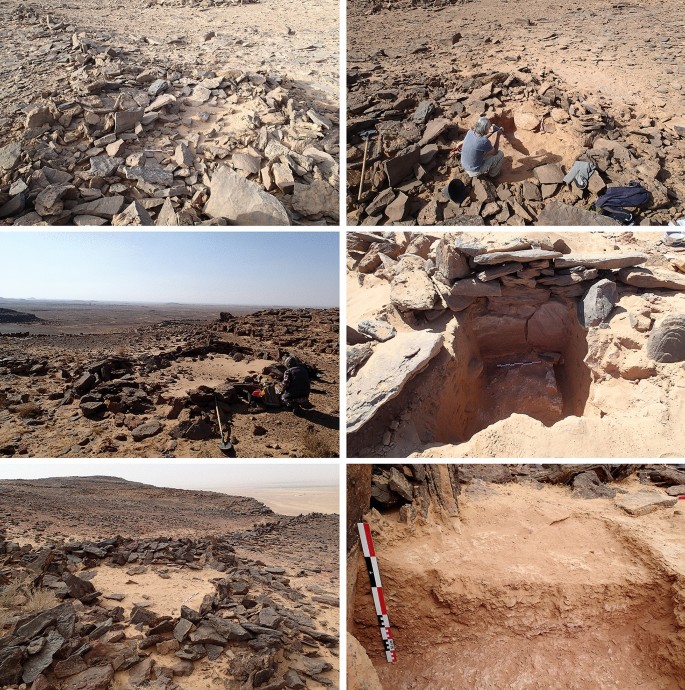The image consists of a grid of six photos arranged in two columns and three rows, each showcasing an outdoor scene of an excavation site. The photos predominantly feature rocky terrain under a clear blue sky. In the middle of the grid, the ground transitions to a smoother surface with rings of darker-colored rocks that contrast with the surrounding lighter soil. A noticeable feature of the top right photo is a person, possibly a female, dressed in tan pants and a blue shirt, using a brush or similar tool, likely for excavation purposes. A blue coat is casually placed on the rocks nearby. The bottom right photo includes a stick, or measuring rod, characterized by black, white, and red alternating bands. A sign with similar colors is also visible, indicating some form of markings or instructions related to the excavation process. Numerous rocks and sparse human activity suggest an in-depth archaeological or geological survey.